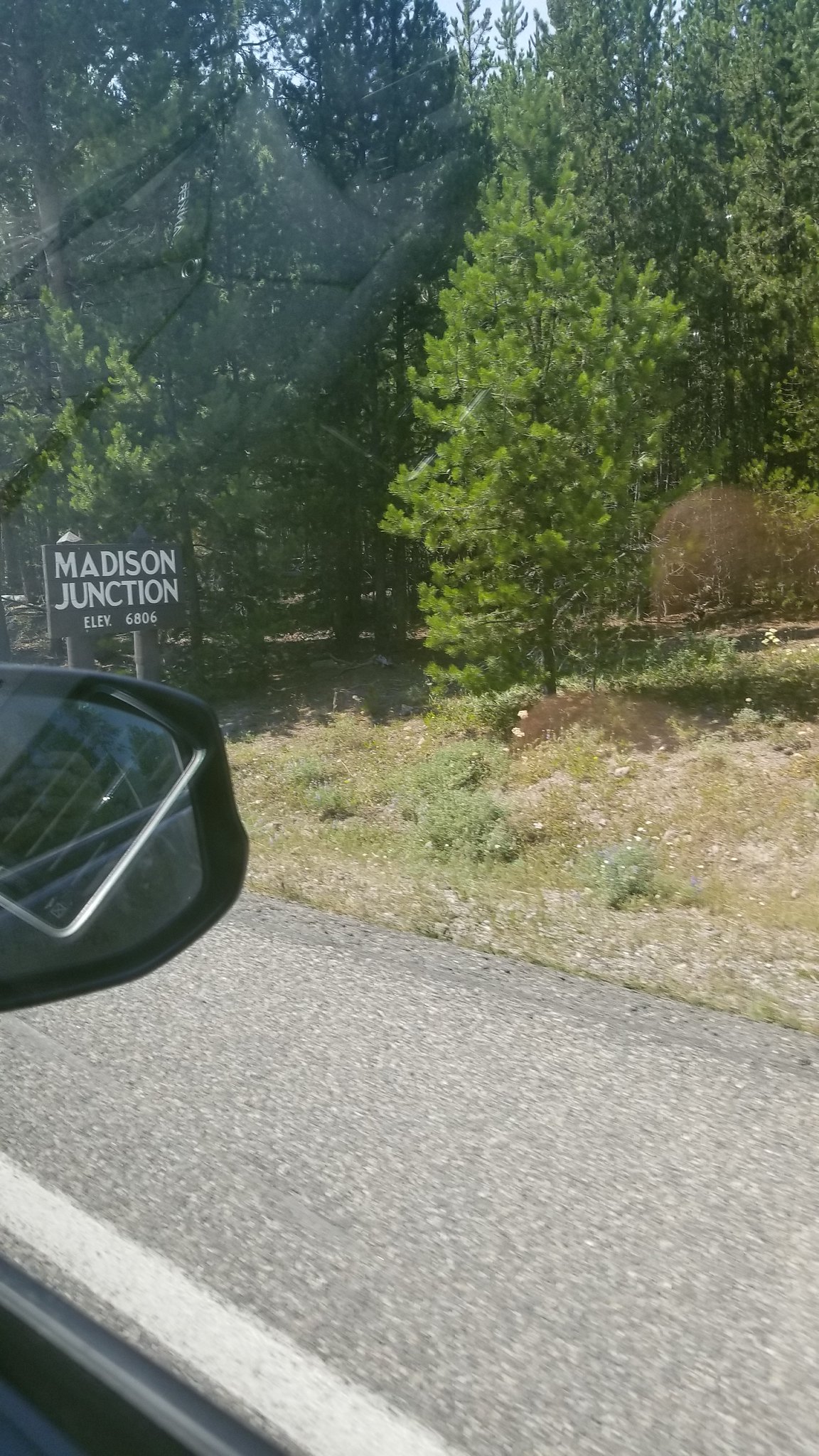The image captures a scene taken from the front passenger seat of a moving vehicle. Prominently, the right-hand side mirror displays part of the vehicle's windowsill and the reflection of the person's knuckles holding the camera. In the background, the photo focuses on a wooden rectangular sign supported by two timber posts, reading "Madison Junction" in white carved letters against a dark backdrop, with "ELEV. 6806" noted below. The sign is set amidst a landscape featuring craggy brown grass and an array of dark to medium green evergreen trees. The road beside the vehicle has a visible white shoulder line marking the boundary between the lane and the concrete shoulder. Additionally, subtle reflections of the vehicle's air conditioning vent and dashboard are discernible on the window glass.